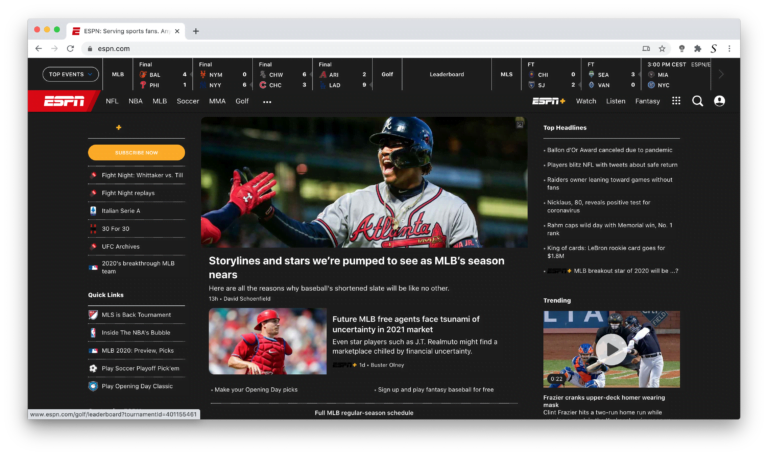**Detailed Caption:**

The image is a screenshot of the ESPN.com homepage as viewed on a computer. At the very top, the URL bar displays "ESPN.com." Directly below the URL bar, the ESPN logo is prominently featured on the left-hand side. The logo consists of the bold, uppercase letters "E," "S," "P," and "N" in white, encased in a red rectangular semi-box with distinctive line work through the text.

The main body of the webpage is divided into several sections. In the center, there is a feature article focusing on Major League Baseball (MLB). This section highlights an image of an Atlanta Braves player engaged in a high-five, capturing a moment of camaraderie. Right below the image, a headline reads, "Storylines and stars we're pumped to see as MLB season nears," suggesting excitement and anticipation for the upcoming season. This central column is densely packed with various news articles and updates related to current sports events.

To the right of the central feature, a sidebar lists the top headlines of the day, complete with links for easy access to full articles. Beneath this is a "Trending" section, which includes a video thumbnail with a play button overlay, hinting at popular or viral sports videos currently circulating.

On the far left, towards the bottom of the page, there are quick links providing easy navigation to other parts of the ESPN website, offering users an organized and user-friendly web experience.